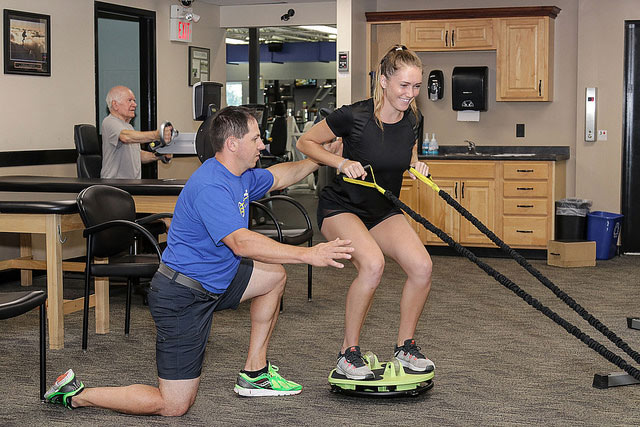In this detailed, color photograph showcasing a scene of physical therapy, a young, blonde, Caucasian woman is central to the image, actively standing on a neon green balance board inside a fitness or rehabilitation room. She is dressed in athletic gear, including a black polyester T-shirt, black shorts, and gray sneakers. With her body slightly bent forward, she is engaging with black elastic straps that have yellow handles, pulling them tightly from the right side for resistance.

Beside her, a Caucasian man, presumably her coach, is kneeling on one knee with the other knee bent. He is ready to support her balance, extending his arms to assist. He has short black hair and is outfitted in a blue T-shirt, navy blue shorts with a black belt, and neon green Saucony shoes.

The room itself has carpeted flooring and various equipment indicative of a therapeutic environment. In the background, an elderly man in a gray shirt engages with exercise equipment, possibly monitoring his progress on a screen or using a blood pressure cuff. Behind this scene, oak cabinetry with a sink is visible as part of a kitchenette setup, along with several tables and chairs. To the far back, an open door leads to the main gym area, further emphasizing the room's functional, clinical setting in a landscape orientation composition.